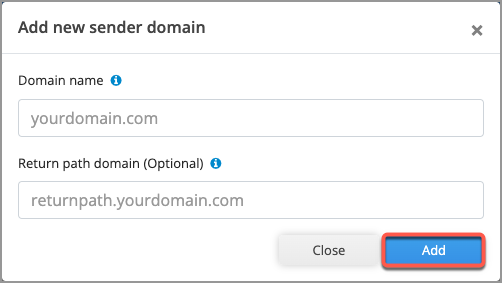This image depicts a user interface on a webpage for adding a new sender domain. At the top, the header reads "Add New Sender Domain." Below this, there is a labeled input field for "Domain Name," where users are instructed to enter their domain name, typified as "yourdomain.com". Beneath this is an optional field labeled "Return Path Domain (Optional)," where the placeholder text is "returnpath.yourdomain.com". At the bottom of the interface, two buttons are visible: one labeled "Close" to exit the process, and another labeled "Add" to submit the information.